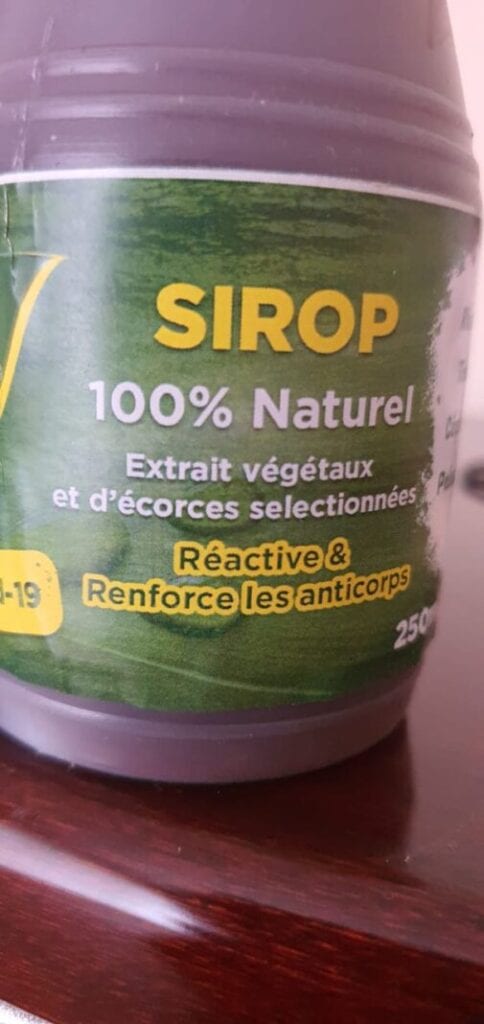The image is a close-up photograph of a plastic bottle of syrup positioned slightly cut-off at the top on a dark, shiny, wooden surface. The scene appears to be indoors, likely in a kitchen. The bottle features a semi-transparent label adorned with a design reminiscent of a green watermelon pattern. This label prominently displays the text "Sirops 100% Naturel Extrait Vegetaux" in yellow and white, indicating a natural extract syrup, with some words possibly being French. There are two horizontal ridges above the label. Inside the bottle, a liquid can be seen. The bottom right corner of the label has the number 250 in white, and the bottom left corner has the number 19 inside a gold rectangle. The overall color scheme includes brown, green, yellow, and white. Light reflecting off the surface adds a touch of brightness to the scene.